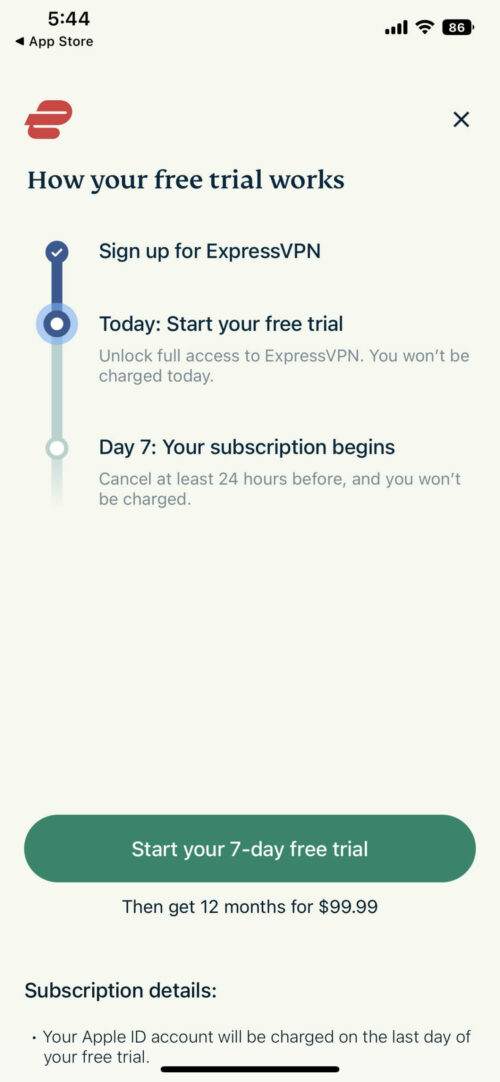The image appears to be a screenshot of a mobile phone screen featuring a promotional page for ExpressVPN. 

- At the very top left corner, "5:44" is shown, likely indicating the time.
- Directly below the time, there's a left arrow icon and "App Store" is mentioned on the right side.
- The top-right corner displays icons for cellular signal strength, Wi-Fi connectivity, and an 86% battery indicator.

Beneath these icons, there is a prominent red, stylized lowercase "e" on the left side, next to an "X" on the right, potentially representing the ExpressVPN logo and a close button, respectively.

A heading below this reads: "How Your Free Trial Works," followed by a vertically-oriented line dividing the section into three parts, each highlighted with a circular icon.

1. The first circle at the top is blue with a white checkmark inside, labeled "Sign Up for ExpressVPN."
2. The second circle below it is blue with a white center and details: "Start Today. Start your free trial. Unlock full access to ExpressVPN. You won't be charged today."
3. The third circle at the bottom is light blue with a white center, providing further details: "Day 7 Your subscription begins. Cancel at least 24 hours before and you won't be charged."

The background color of the sections is a mix of white and off-white. 

At the bottom of the image, there is a very large green button, spanning the width of the screen. The button has the text in white: "Start Your 7-Day Free Trial." Below this button, it mentions a subscription offer: "Get 12 months for $99.99."

Repeatedly, below everything, it emphasizes: "Start Your 7-Day Free Trial," rendering the promotion unmistakably clear.